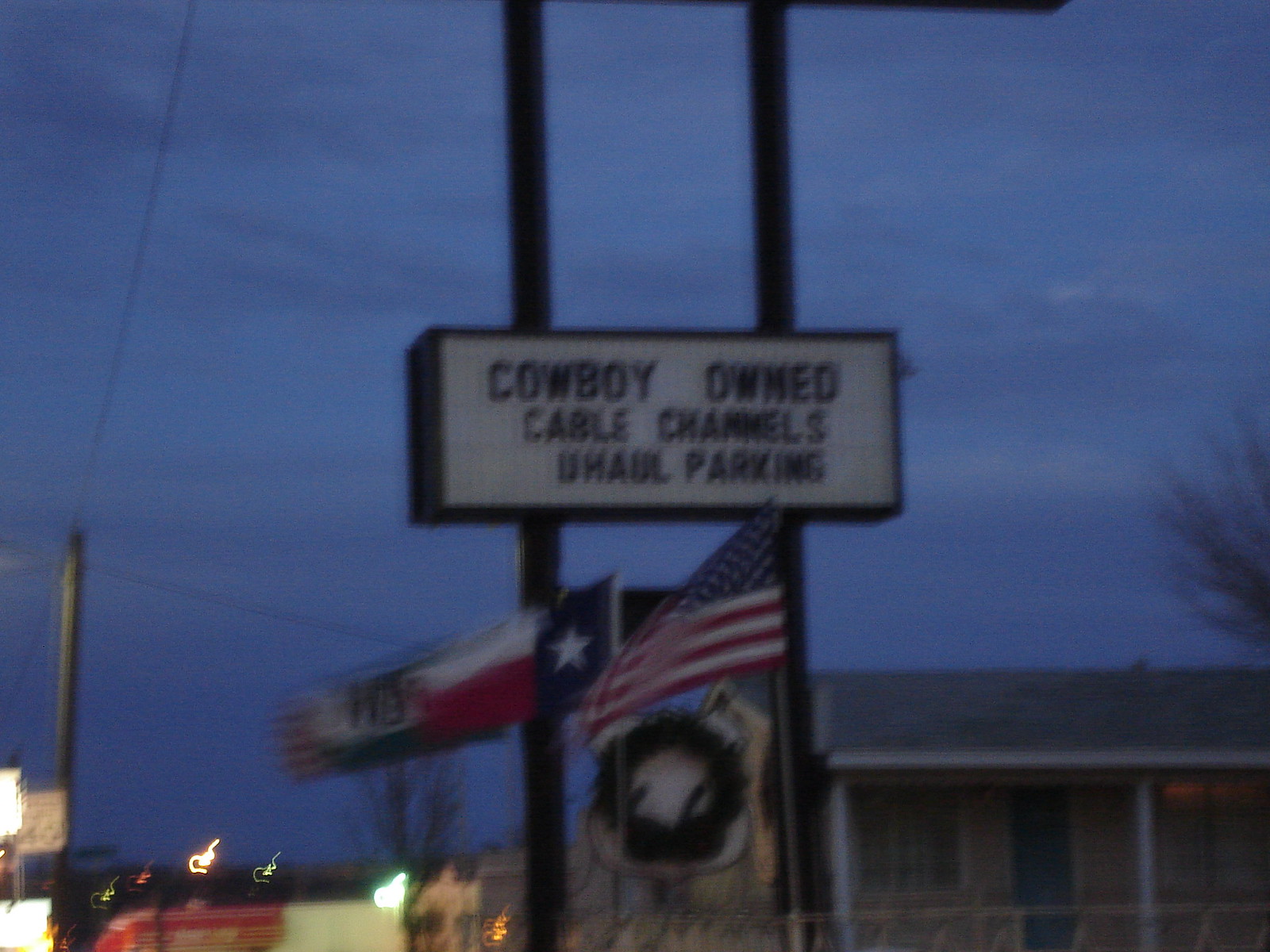The photograph captures a nighttime or evening scene with a dark blue sky interspersed with dark blue and white clouds. In the distance, various lights and billboards are visible, though some of them are cut off. A large, gray pole with lines extending from it is also present, adding to the urban atmosphere. The focal point of the image is a brown building with white pillars supporting a gray roof and a white overhang, likely a motel based on other visual cues.

Dominating the center of the image is a large, rectangular white sign, outlined in black and held up by two black poles. The sign features all-capital black lettering that reads "Cowboy Owned," followed by "Cable Channels," and "U-Haul Parking." Below the sign, multiple flags flutter, including a clearly visible American flag and another flag portraying a blue field with a white star, alongside red and white stripes, representing Texas. There are additional flags partially obscured, including one with black text on a white and dark green background and another unidentified flag.

The overall scene includes elements such as utility poles with wires and other blurry details that suggest a bustling, yet slightly faded urban environment. The combination of the building, sign, and flags suggests a quintessential roadside setting, possibly near a motel or a similar establishment.